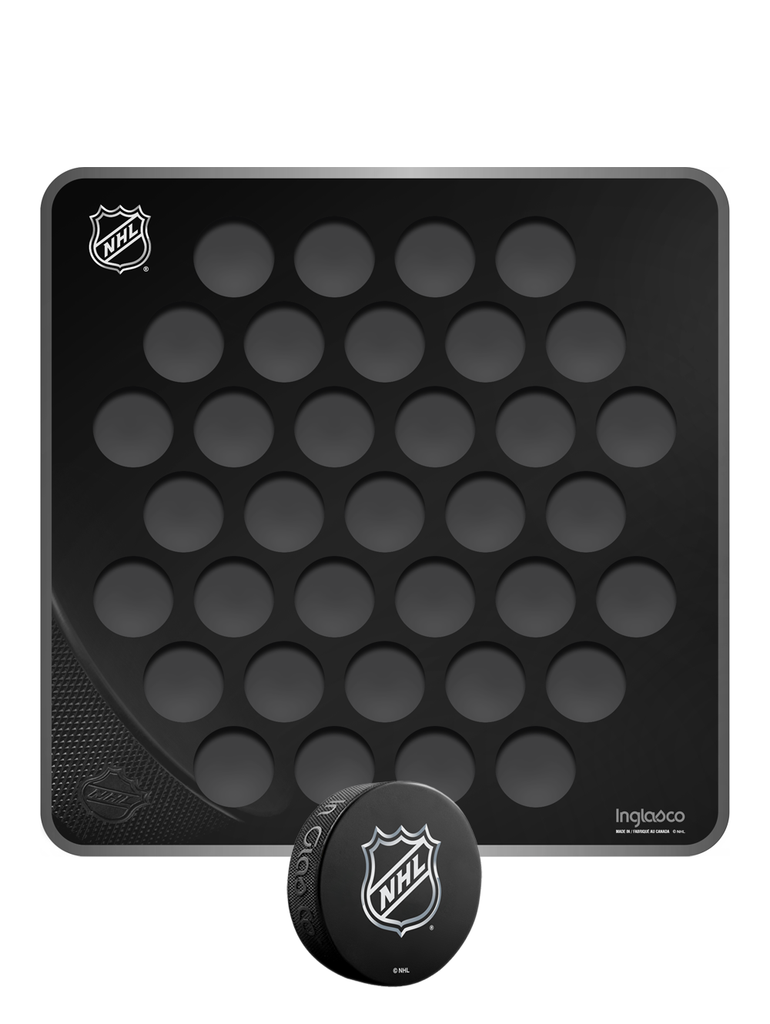This image shows a black, square-shaped object made of plastic, designed to hold hockey pucks. The object prominently features the NHL (National Hockey League) logo in white on the upper left corner. The surface is marked with approximately 30 indented circles, each matching the size, depth, and general dimensions of a standard hockey puck. These indentations are slightly lighter in a blackish-gray shade, creating a subtle contrast against the predominantly black structure. Additionally, the object includes a textured area on the bottom left and a nearly unreadable brand name in gray lettering located at the bottom right. At the bottom of the image, there is a hockey puck adorned with the NHL logo, similar to the one on the holder. The overall design elements and color scheme are limited to black, white, and gray.